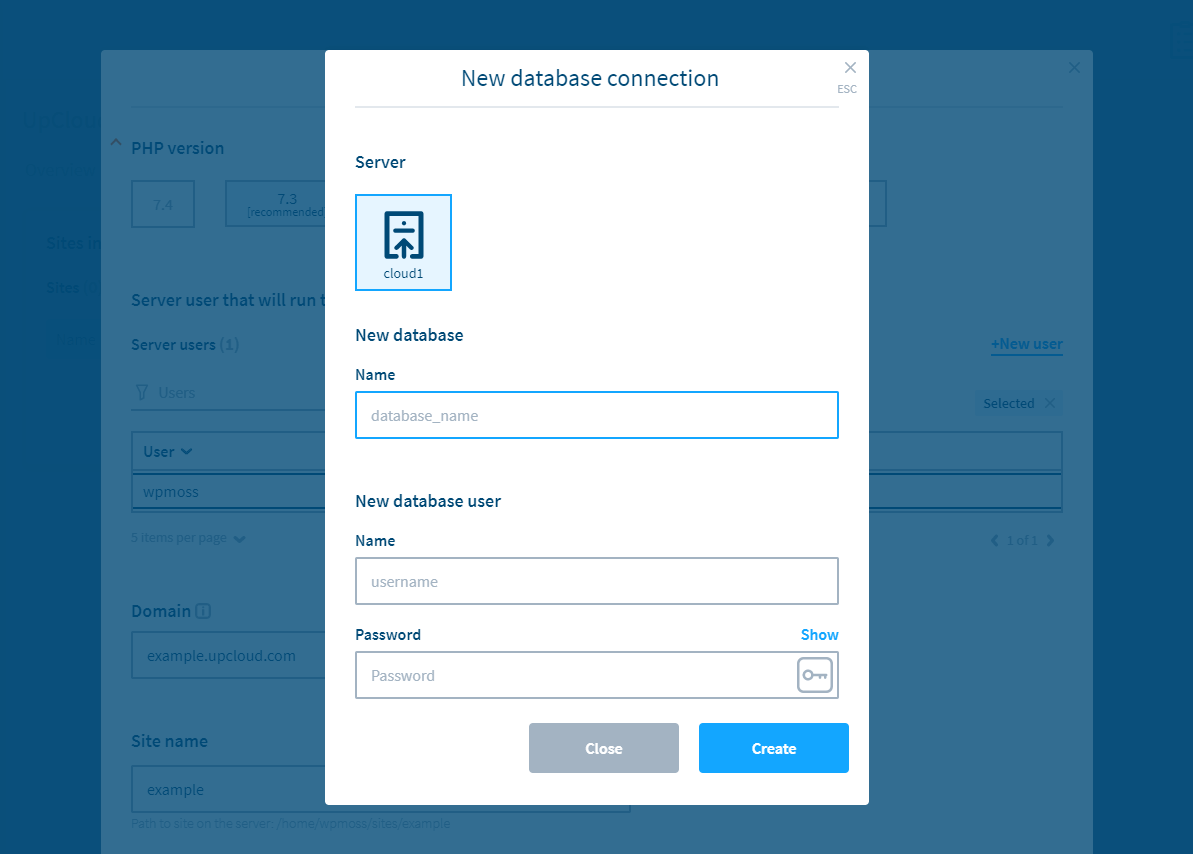The image depicts a digital interface centered around database management. The background is a dark blue screen that is largely obscured by a prominent white rectangular box in the middle of the screen. At the top of this box, the text "New Database Connection, Server" is displayed.

Beneath this heading is a light blue square with a darker blue border. Within this square, there is a graphical icon displaying a piece of paper with a dot at the top and a horizontal line beneath it, from which an arrow points upwards from the bottom of the box. This icon is labeled "Cloud One."

Below this light blue square, the box includes various labeled fields for database setup. The first field is labeled "New Database Name," and presents the placeholder text "DATABASE_NAME." The subsequent field asks for the "New Database User Name," followed by another field requiring a "Username." Next is a "Password" field, followed by a "Show" option to display the entered password.

To the right of the password field, there is a small square containing an icon of a key. 

At the bottom of this interface, a gray rectangular button labeled "Close" and a blue rectangular button labeled "Create" are positioned side by side, offering options to either close the form or proceed with creating the new database.

The background does not offer any discernible details, as it is mostly hidden by the central white box. Notably, there are no depictions of people, animals, plants, flowers, or trees in this image.